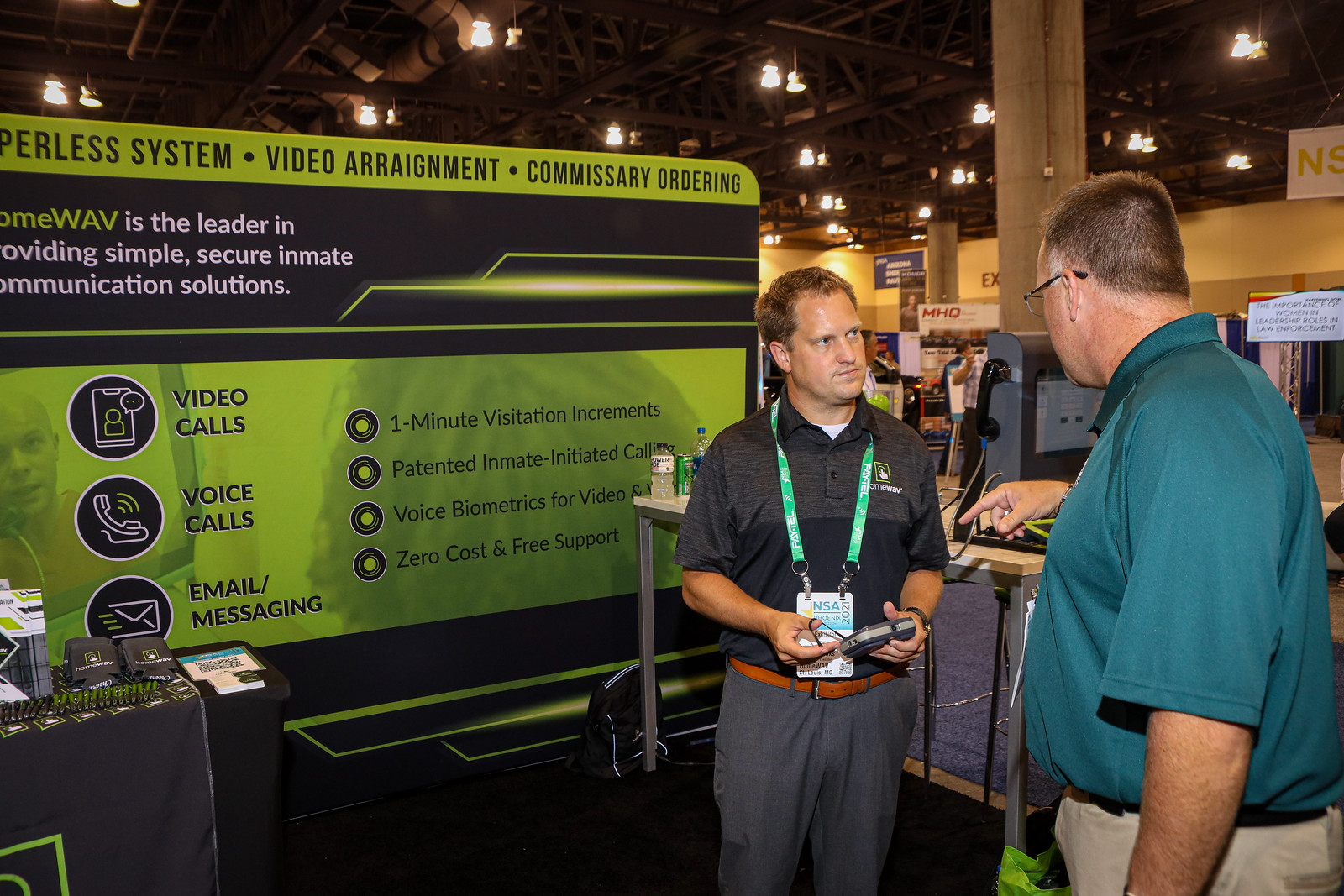In this image, taken at a tech convention or trade show, two men are engaged in a conversation in front of a vibrant lime green and black backdrop. The man on the left, wearing a black collared shirt, grey slacks, and a brown belt, has a lanyard around his neck, likely displaying his name and company details. The other man, standing to his right, is dressed in a green collared shirt and khaki pants, also sporting a lanyard. Both appear to be representatives discussing a video call system that the backdrop prominently highlights.

The backdrop is covered with various elements and details about the product. It features icons representing a cell phone, an old-school phone, and an email message, emphasizing the system's comprehensive communication capabilities including video calls, voice calls, and email messaging. Additional text on the backdrop mentions features such as "video arraignment," "commissary ordering," "one-minute visitation increments," "patented inmate-initiated calling," "voice biometrics for video," "zero cost," and "free support." The backdrop also displays the company name, "HomeWAV."